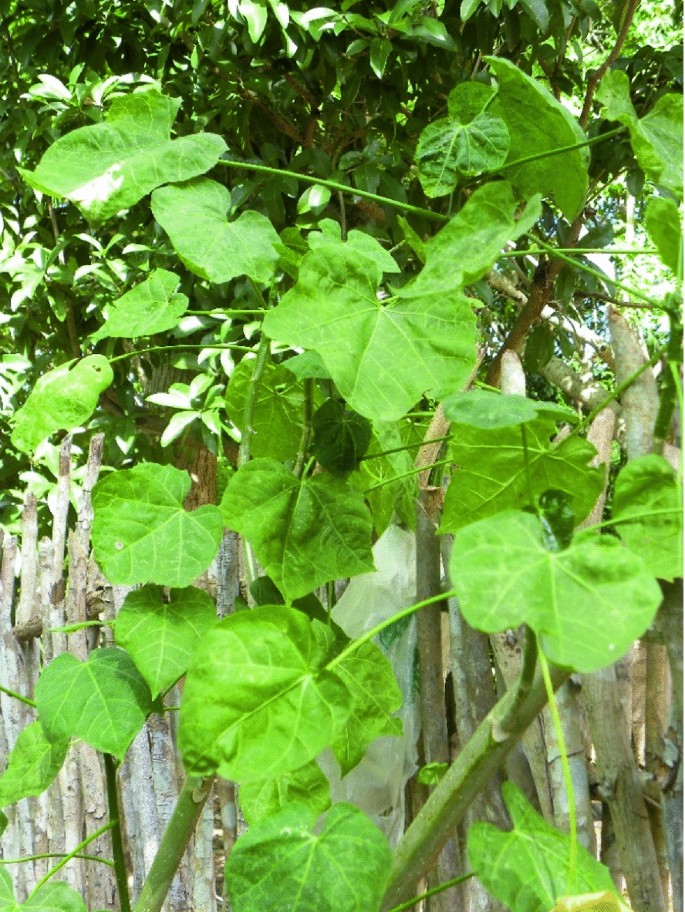The image showcases a lush and vibrant garden scene with various plant life. In the foreground, there is a stocky vegetable-like plant resembling a squash, featuring large, matte, heart-shaped leaves with numerous light yellow-green veins and a rippled texture. These leaves extend towards the camera on stringy stems and are notable for their broad, bright green appearance. Behind this plant, a natural fence composed of vertically stacked sticks creates a visual separation. The rustic fence is constructed from sticks that appear to be broken off and set into the ground, offering a unique, homemade look. In the background, a tree with glossy, dark green, pointed leaves can be seen, adding depth to the image. The scene is brightly illuminated by the sun, which creates a lively and natural ambiance, though the dense greenery provides some shading within the photograph. The overall composition is rich with botanical elements and natural textures, encapsulating a serene and verdant setting.